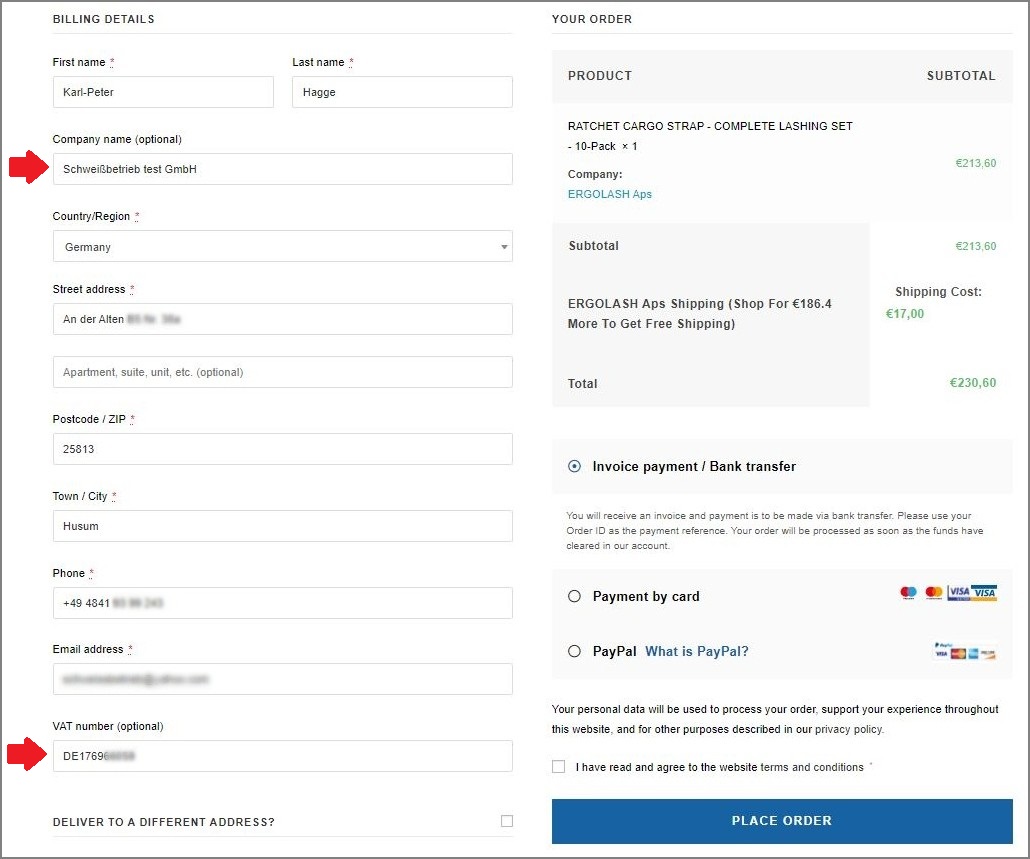A cropped screenshot of an order page on a website with a clean white background. At the top left, the section "Billing Details" is displayed prominently, separated from the form by a gray line. Below this line, fields for "First Name" and "Last Name" are provided, followed by a text box for the optional "Company Name," highlighted by a red arrow pointing at the input field. The "Company Name" box contains an example entry. Further down, fields for "Country/Region," "Street Address," "Postal Code," "Town," "Phone," "Email," and an optional "VAT Number" are displayed. Another red arrow directs attention to the VAT Number field, which contains a partially pixelated number just like the email, phone, and street address fields to ensure privacy.

On the right side of the form, the "Your Order" section starts with a large gray box labeled "Product" and "Subtotal." The detailed product listing reads "Ratchet Cargo Strap, Complete Lashing Set, 10-pack times 1," with the corresponding subtotal shown to the right. Below this, the manufacturer's name is mentioned, followed by another highlight box for "Subtotal" and its amount. Shipping costs are itemized below the subtotal, and the total amount due is listed clearly on the right.

At the bottom right corner, payment options are listed: "Invoice Payment," "Bank Transfer," and "Payment by Card or PayPal." Below these, a checkbox for agreeing to the site's terms and conditions remains unchecked. The section concludes with a prominent blue "Place Order" button.